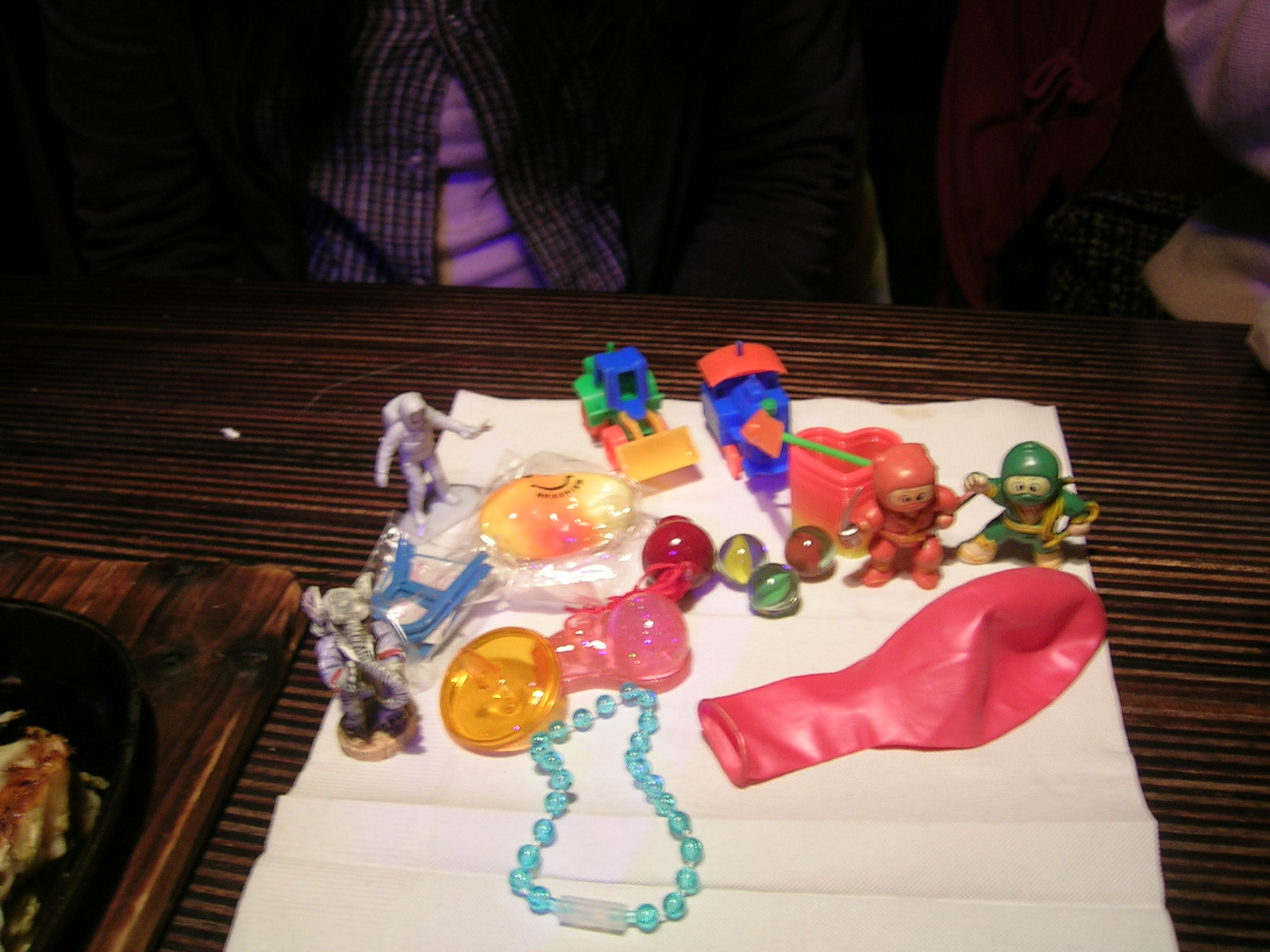The photograph captures a diverse assortment of children's toys and objects meticulously arranged on a piece of white fabric or paper, spread out on a wooden table. Notably, the collection includes an aqua beaded plastic bracelet, an uninflated pink balloon, an elephant figurine, several marbles, a plastic toy train, and a bulldozer. Additionally, diminutive ninja figures, an astronaut figure, and several other small, unidentifiable toys contribute to the scene's playful chaos.

A yellow spinning top and a blurred, translucent vase with a straw add to the assortment. The background features a person whose face isn't visible, dressed in a lavender-colored t-shirt paired with a dark button-down shirt. They sit behind the table, which is partially bordered by a dark wooden board on the left. The scene encapsulates a playful snapshot of childhood knick-knacks and their varied forms.